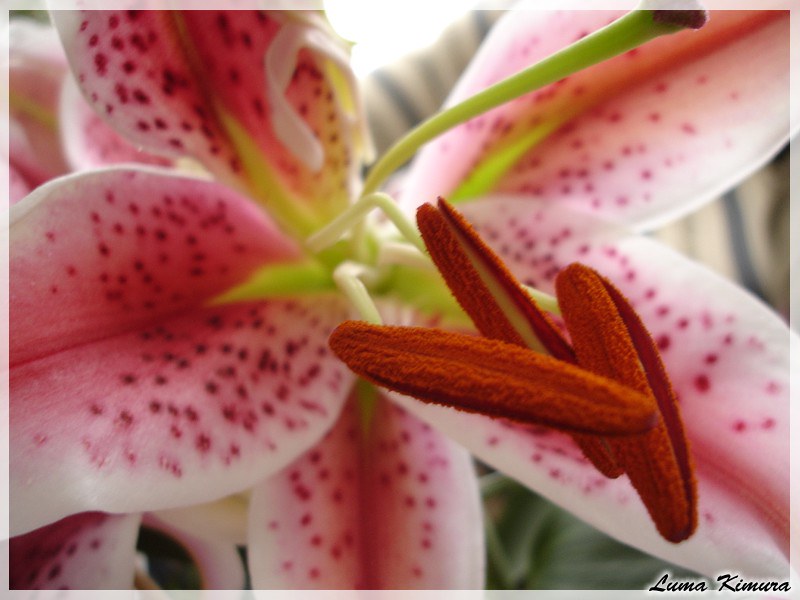This is a detailed, extreme close-up color photograph of a pink daylily captured in landscape orientation. The focus is on the intricate interior of the flower, particularly highlighting its distinct features. The blossom consists of five main petals which exhibit a delicate gradient from light pink to dark pink, with a striking pattern of dark red speckles and a central dark red streak on each petal. The petals are slightly out-of-focus toward the edges, emphasizing the core elements of the flower.

Central to the image are several green filaments, resembling stems and leaves, with three elongated, fuzzy anthers at their tips. These anthers are a deep red color and have an elongated ellipse shape, bearing a resemblance to miniature French bread loaves, with the interior of one appearing yellow.

The background is blurred, featuring indistinct blue and white stripes, likely indicating additional foliage or environmental elements. The bottom right corner of the image bears the signature “Luma Kimura” in black script with a white drop shadow. The photograph is presented in a representational realism style, with a narrow lightened border framing the composition.